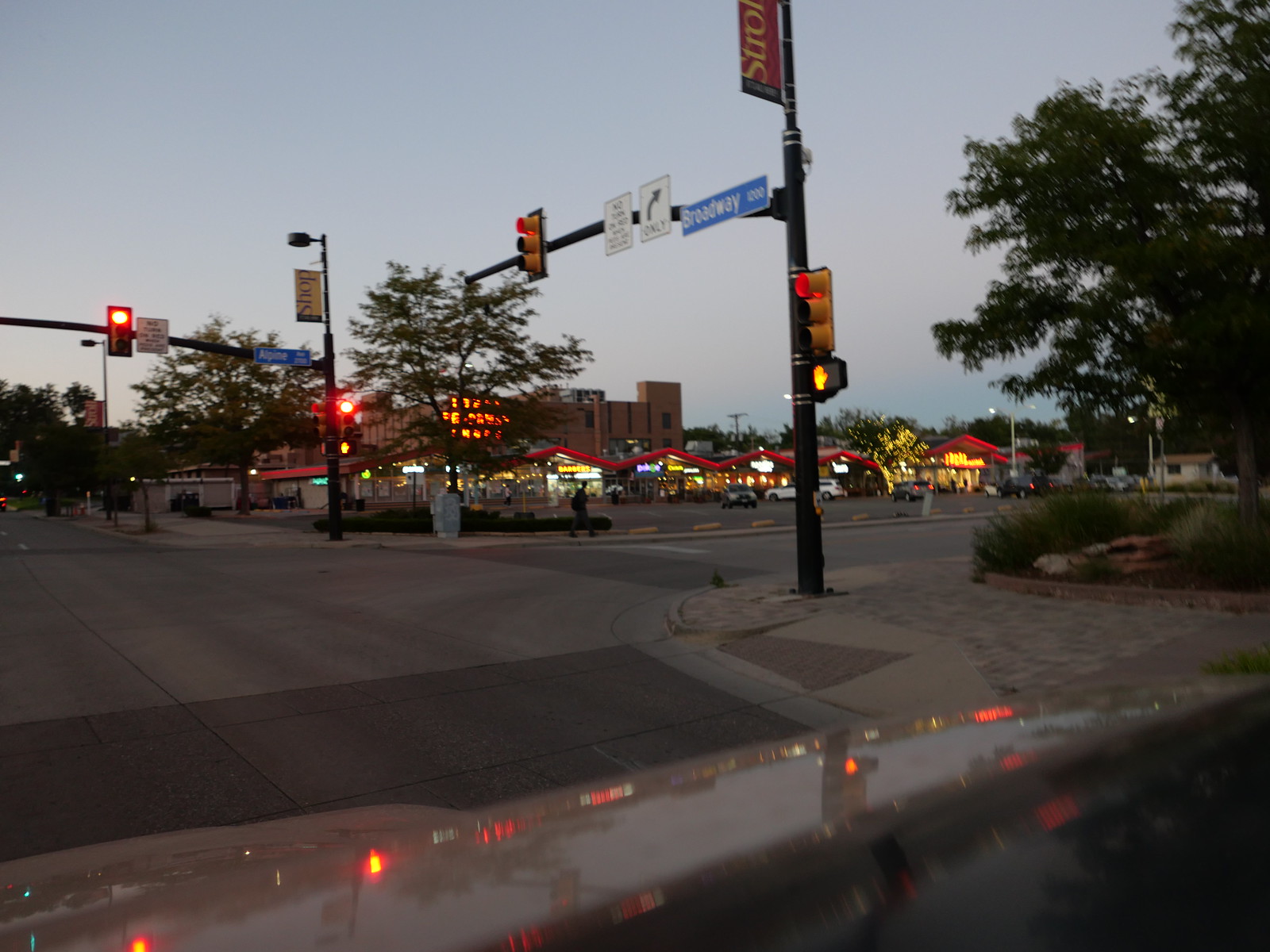This photograph captures a street intersection at dusk, with a bluish-gray sky indicating the late evening hour. In the distance, a shopping center with various businesses and a parking lot with several cars can be seen. The photo is taken from the driver's seat of a car approaching the intersection, where all the traffic lights are red. A street sign reads "Broadway" and "Right Turn Only." Additionally, a tree stands beside the intersection, adding a touch of nature to the urban scene.